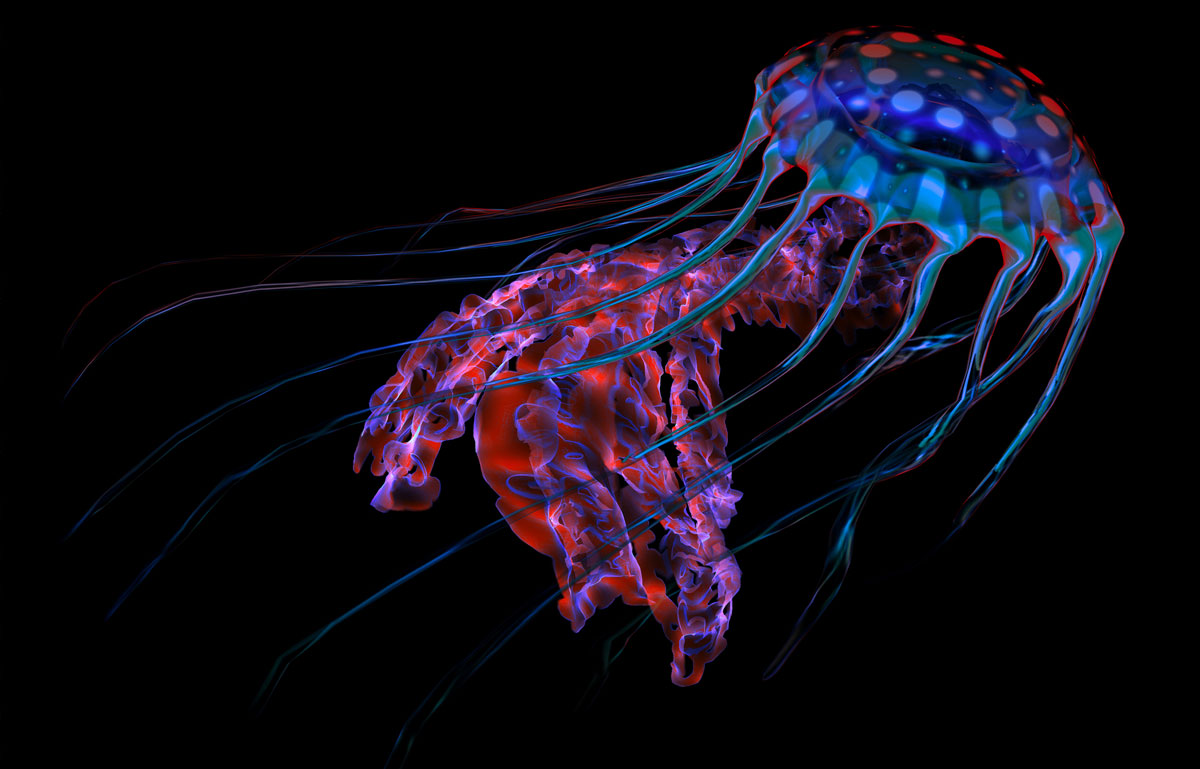In this captivating and vividly detailed image, a jellyfish takes center stage against a stark, all-black background, making its colors stand out brilliantly. The jellyfish is positioned in the top right corner of the image, and its bell or top part shimmers in blue and light blue hues, adorned with scattered red and blue dots. This combination of colors highlights the intricate beauty of the creature. The tentacles, extending gracefully from the bell, exhibit a mesmerizing palette of blues with reddish underglows. Some tentacles appear thicker and merge shades of red, blue, and white, giving them a textured and dynamic look. Additionally, there are pink and purple hues interspersed within the array of tentacles, creating a sense of fluid motion as if the jellyfish is gently flowing through the water. The image, possibly a painting or a highly stylized computer graphic, employs various effects to evoke a sense of depth and realism, capturing the ethereal essence of the jellyfish in its dark aquatic surroundings.